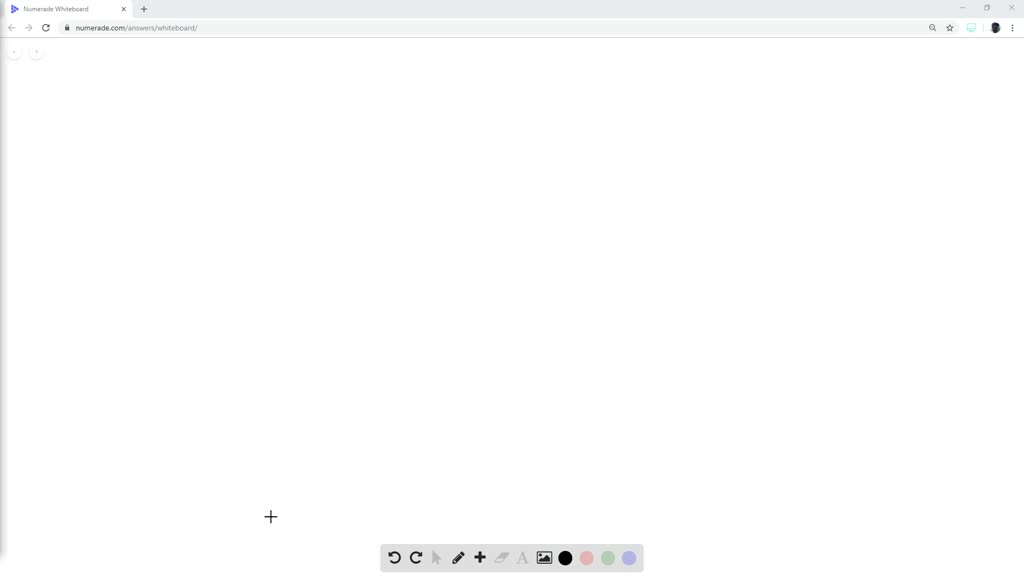The image depicts a digital whiteboard with minimal content. The whiteboard itself is largely blank, save for various arrows and squiggly lines in blue, green, pink, and black, scattered across the surface. There is a small picture placed on the board, accompanied by a plus sign, and a pencil icon. At the bottom of the screen, a toolbar features left and right arrows.

The cursor is represented by another plus sign near the top of the screen. At the very top, a plain gray and tan bar contains directional arrows pointing left and right.

Below this header bar, there is another gray and tan bar with several symbols. On the left side of this bar is an arrow icon and the file name. To the right are additional icons including a star, a magnifying glass, a blue computer screen symbol, and an image resembling a silhouetted face.

In summary, the image is of a sparsely populated digital whiteboard with various colorful annotations and a few toolbar and header icons, suggesting a user interface for drawing or note-taking.